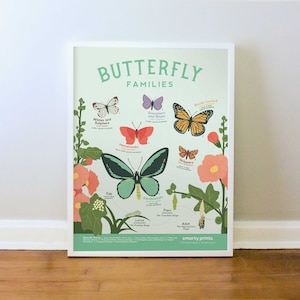This photograph features an art piece set against a clean, light-grayish white wall with a white baseboard, situated on a brown wooden floor. The artwork is framed in a white frame and is titled "Butterfly Families" in light green and blue lettering. The poster captures various colorful cartoon butterflies and flowers against a slightly green-white background that distinguishes it from the wall. Butterflies of multiple colors—such as yellow, light blue with black wings, purple, monarch orange, pinkish red, and a giant green one with a black stripe—are depicted. The piece also portrays flowers, including a vibrant pink flower with a yellow center and green leaves. Despite the small size of the text, it's clear the poster provides information about the different butterflies and possibly details the stages of a butterfly’s lifecycle, including eggs, caterpillar phases, and cocoon to hatching stages. The image is vibrant and bright, with a clean, catalog-like aesthetic, reminiscent of something you might find on Etsy.